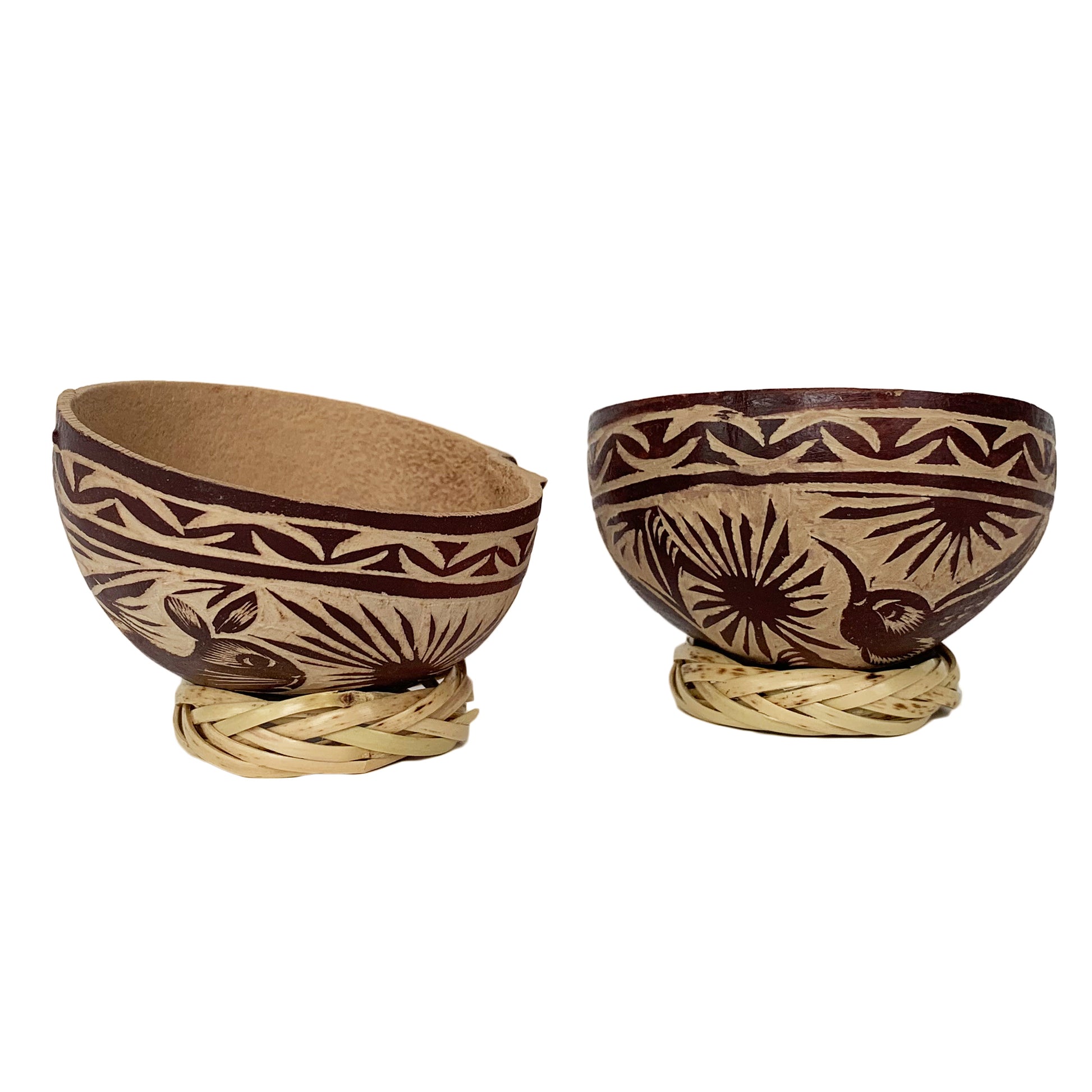This image showcases two modern clay pots with intricate designs, both seated on a bamboo stand. The background is a solid white, suggesting a display setting perhaps for an online sale. Each pot, rendered in light brown clay with darker brown adornments, features unique Native American-inspired patterns. 

The pot on the right displays a rabbit motif with detailed features—one ear pointing to the left and another upward, a vivid brown eye, and streaks decorating its face. Surrounding the rabbit is a circular pattern reminiscent of sunrays.

The pot on the left carries a similar design theme but highlights a bird instead. The bird is depicted with a pronounced beak stretching up and to the left, and a tail curving upward to the right. Its eye is also brown, accentuated by a contrasting white area around it. Both pots share geometric patterns, like triangles and bands, enhancing their visual appeal.

The bamboo stand, crafted from intricately woven wicker lines, provides a natural, artisanal base for the pottery, complementing their earthy tones and adding to their handcrafted aesthetic.